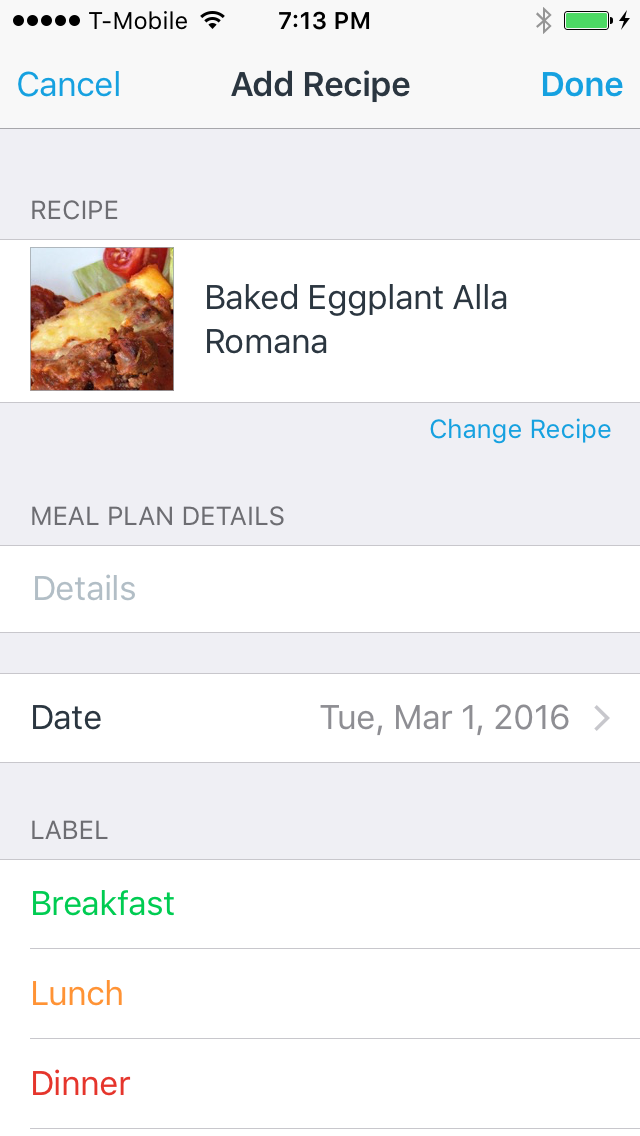In this image, the screen of a smartphone is displayed, showcasing various interface elements. 

- In the top-left corner, there is a connection bar with 5 out of 5 dots indicating full signal strength, accompanied by the network name "T-Mobile" and a Wi-Fi icon.
- At the center of the top bar, the time "7:13 PM" is written in black text.
- On the top-right corner, a battery icon shows full charge.

Below this bar, there are three options aligned horizontally:
- "Cancel" written in light blue text on the left.
- "Add Recipe" in black text at the center.
- "Done" in blue text on the right.

The main section of the screen features a recipe interface:
- A gray section with the title "Recipe."
- Below this, on a white background, there is an image of food labeled "Baked Eggplant A La Romana."

Further details are provided in the subsequent sections:
- Another gray section at the top right states "Change Recipe" in blue text.
- The bottom left of the gray section reads "Meal Plan Details."

Below this:
- Another white background section indicates "Details."
- This is followed by additional gray and white sections displaying specific information:
  - A date labeled "Tuesday, March 1st, 2016."
- Subsequently, a gray section is labeled "Label," followed by a breakdown of meals listed in colored text:
  - "Breakfast" in green.
  - "Lunch" in orange.
  - "Dinner" in red.

This detailed layout captures the complete interface of the smartphone screen, offering a clear view of the recipe and meal planning details from top to bottom.